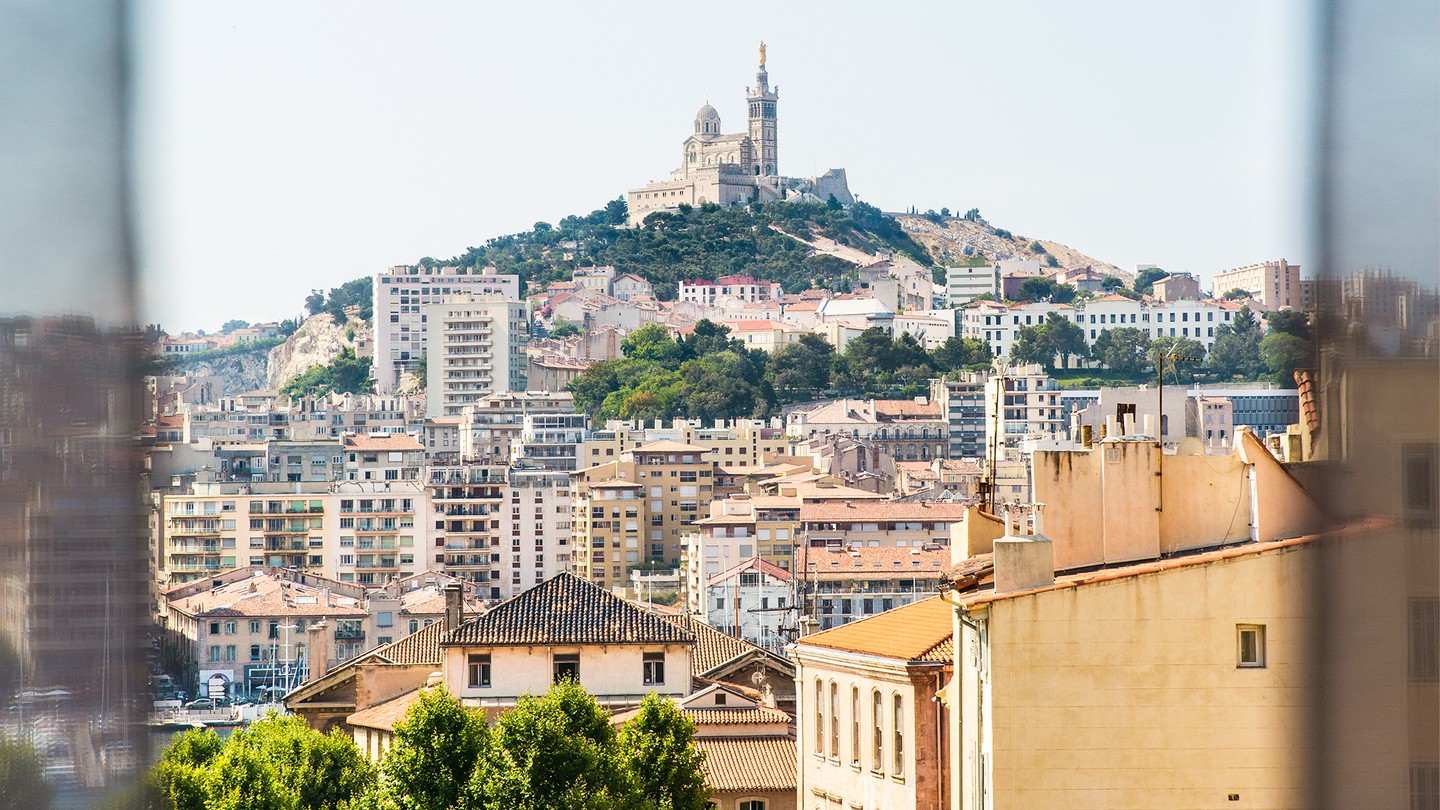This photograph, taken from indoors as evidenced by the visible curtains framing the shot, captures a densely built terraced town sprawling across a hillside. The foreground is dominated by an array of closely clustered, multi-storied buildings, primarily painted in beige or white and topped with reddish roofs. These buildings, ranging from three to ten stories, exhibit a classic European architectural style and appear quite old, with some emitting a yellowish hue under the sunny light, although the sky itself is not particularly vivid.

The town extends up the hillside, which is interspersed with large patches of green trees. The buildings are terraced at various levels, creating a cascading effect up the hill. At the apex of this terraced arrangement stands a substantial and historic-looking structure with numerous wings. This monumental structure features a dome on one end and a turret or tower on the other, adorned with an impressive golden sculpture, suggesting it could be a significant church, mosque, or other religious edifice. The photograph strategically highlights the contrast between the densely packed urban area and the verdant hillside, offering a comprehensive view of this picturesque town.